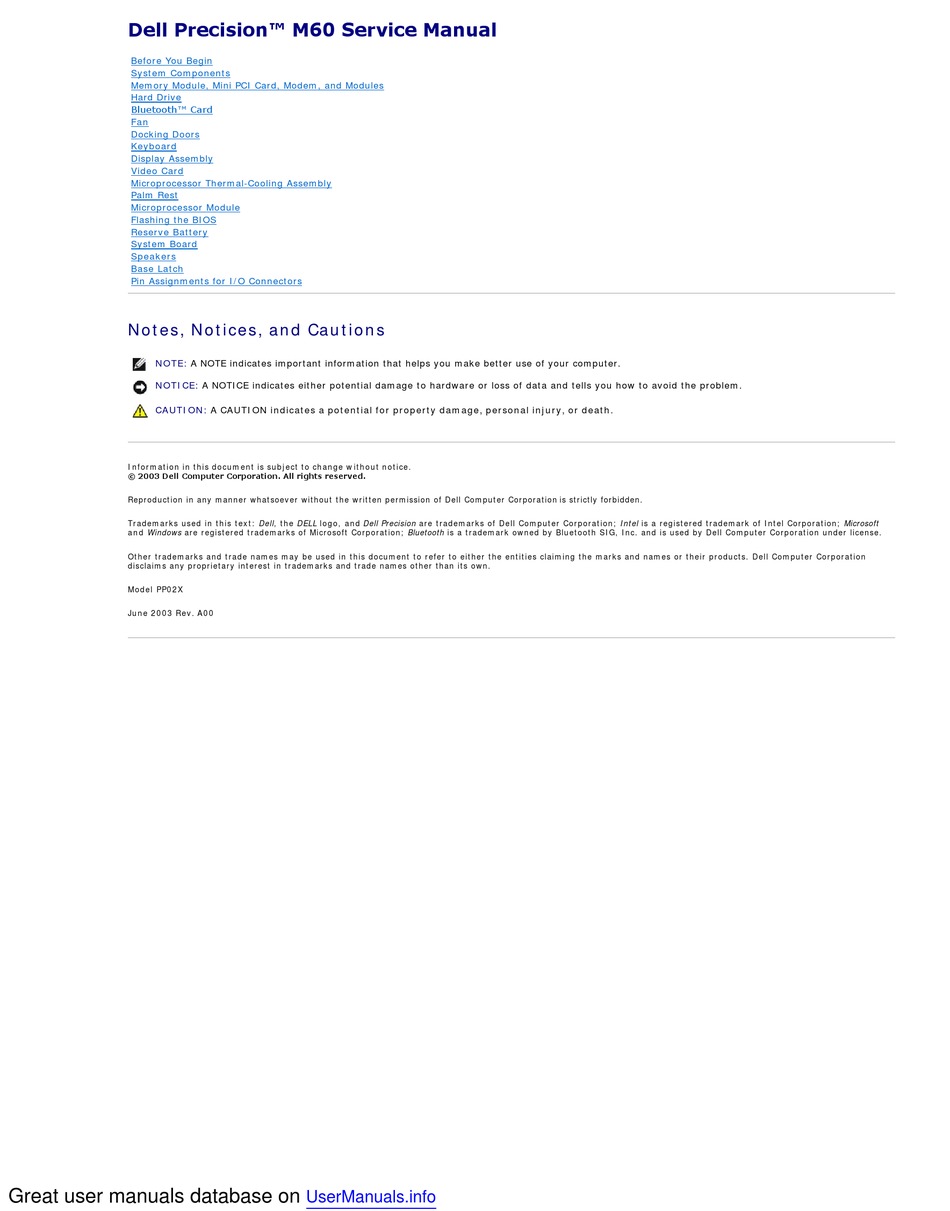The image displays a detailed page from a Dell Precision M60 Service Manual. At the top in blue font, it reads, "Dell Precision™ M60 Service Manual." The manual features a comprehensive table of contents with light blue hyperlinks. Key sections include "Before You Begin," "System Components," and subsections such as "Memory Module," "Mini PCI Card," "Modem and Modules," "Hard Drive," "Bluetooth Card," "Fan," "Docking Doors," "Keyboard," "Display Assembly," "Video Card," "Microprocessor," "Thermal Cooling Assembly," "Palm Rest," "Microprocessor Module," "Flashing the BIOS," "Preserved Battery," "System Board," "Speakers," "Base Latch," and "Pin Assignment for I-O Connectors."

Noteworthy information boxes are also highlighted:
- **Note:** Indicates important information to optimize computer use.
- **Notice:** Warns of potential hardware damage or data loss and provides preventive measures.
- **Caution:** Alerts to the potential risks of property damage, personal injury, or death.

The document states that its information is subject to change without notice and is copyrighted by Dell Computer Corporation in 2003, with all rights reserved.